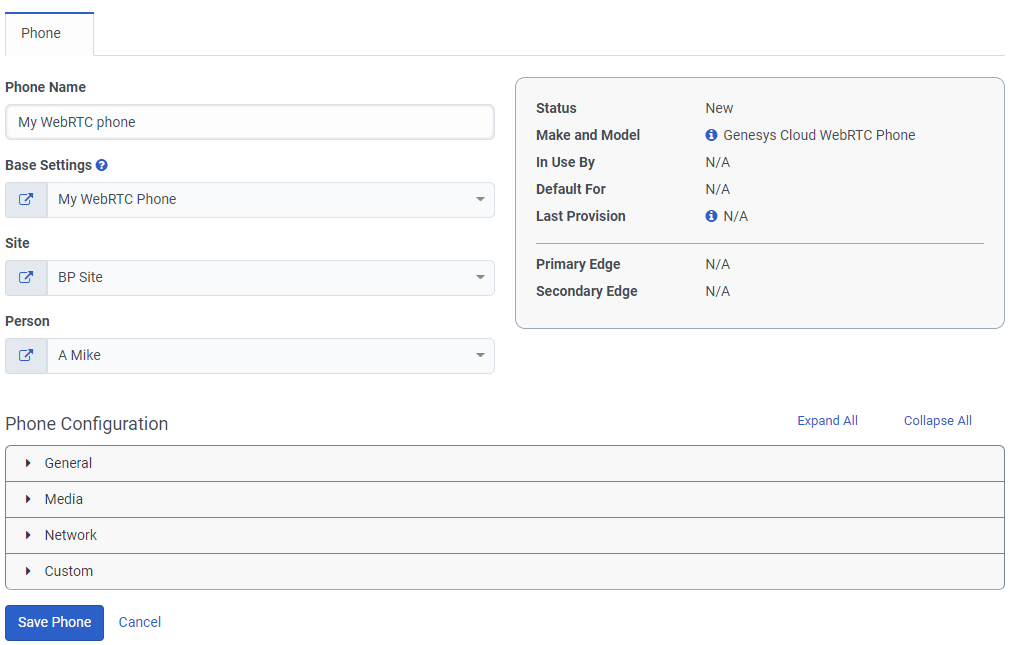The image depicts a detailed web page interface designed for adding and configuring a phone. At the top, there is a tab labeled "Phone". Below this, there is a text box prompting the user to enter the phone name. The section that follows is titled "Base Settings" with an adjacent question mark icon for additional information. The first setting is a dropdown menu labeled "My WBRTC Phone". Next, there is an option labeled "Site" with a dropdown menu and an additional link indicating that it can be opened in a new window. Further down, there is another dropdown menu labeled "BP Site".

On the right side of each dropdown menu, there is an icon resembling a microphone and another dropdown arrow. Adjacent to these settings, there is a status box displaying: "Status: New", "Make & Model: Genesis Cloud Web RGC Phone", "Used by: NA", "Default for: NA", "Last Provision: NA", "Primary Age: NA", and "Secondary Age: NA".

At the bottom of this section, there is a heading "Phone Configuration" with options to "Expand All" or "Collapse All". Four distinct sections are available for configuration, represented by boxes with forward, left-facing, and right-facing arrows. These sections are labeled: "General", "Media", "Network", and "Custom".

Finally, at the bottom of the page, there are two buttons: one to "Save Phone" and another to "Cancel". The overall layout suggests an interface for listing and configuring phone settings with options to save or cancel the changes.